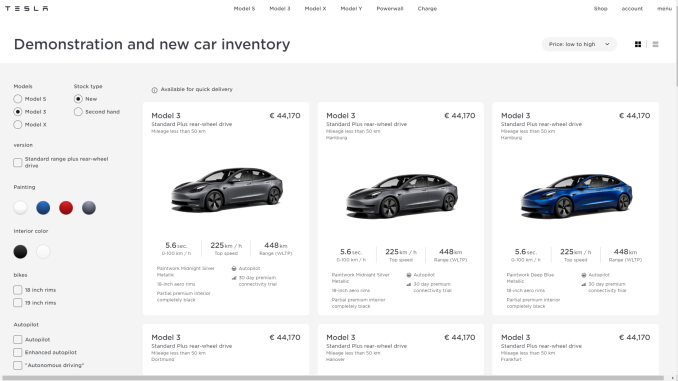The image depicts a webpage displaying a selection of Tesla Model 3 vehicles from the Demonstration and New Car Inventory section. The background of the page is predominantly white. At the top of the page, there are navigation options for Model S, Model X, Model Y, Powerwall, Charge, Shop, Account, and Menu. The cars are currently sorted by price in ascending order.

Three Model 3 vehicles are visible on the screen, each listed at a price of 44,170 Euros. Specifications mentioned on the page include a top speed of 125 kilometers per hour and a range of 448 kilometers, all provided in kilometers. The three vehicles primarily differ in color. One car is a dark gray, another is a slightly lighter gray, and the final one is blue. Some of the features and finer details are not fully legible in the image.